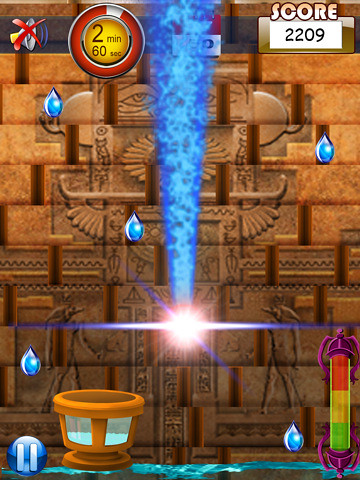This image appears to be a screenshot from a video game, possibly an app available on both mobile and computer platforms. The scene is set inside a pyramid, characterized by its distinct architectural style and hieroglyphic symbols commonly associated with ancient Egypt. The walls are adorned with depictions of people and symbols reminiscent of those seen in historical pyramid interiors. Additionally, there are small, blue droplets resembling water falling from the top of the screen. A timer is displayed at the top, currently reading 2 minutes and 60 seconds, while the player's score stands at 2209.